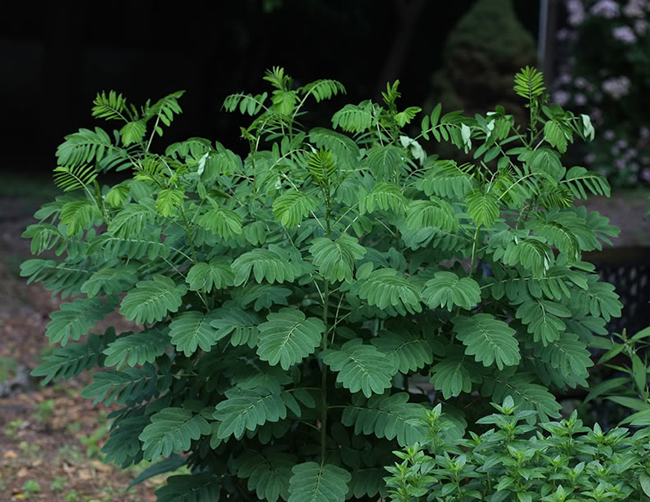The photograph captures a garden scene focused on a large fern or a group of ferns with typical green leaves. Some leaves are a brighter green, possibly indicating new growth. The scene is set outdoors under a gray, overcast sky, resulting in diffuse lighting that gently illuminates the greenery. The fern has numerous stems, numbering around three dozen, creating a dense, bush-like appearance. In the lower right corner of the image, another plant is growing, and the bottom left reveals exposed soil. The background features additional greenery and some pink flowers in the upper right, along with a pole partially visible. The overall setting is a garden, grounded in the natural texture of dirt and framed by a subdued and evenly lit environment.